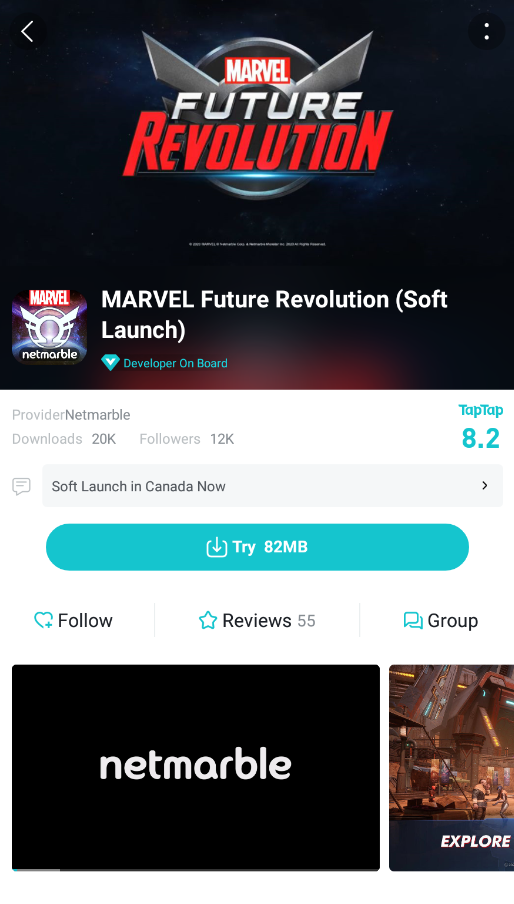**Marvel Future Revolution** - App Store Page

At the top of the page, a vibrant banner prominently displays the game title "Marvel Future Revolution" in bold, red letters, accompanied by a striking shield icon with wings. The background features a dark, space-themed design, adding to the game's epic feel. Below the title, the text "Marvel Future Revolution soft launch" is highlighted in red, with the iconic Marvel logo to the left of the shield icon, and the developer name "Netmarble" below it.

Under this section, there is detailed information about the developer and the game's performance metrics. The entry reads:
- **Developer**: Netmarble
- **Downloads**: 20k
- **Followers**: 12k
- **TapTap Rating**: 8.2 (in a teal color)

A notification indicates that the game is currently in a soft launch phase in Canada. A greenish-blue "Try" button shows the download size of 82 megabytes. Additional options include:
- **Follow**: Indicated by a heart icon
- **Review**: Indicated by a star icon with a count of 55 reviews
- **Group**: Represented by greenish-blue bubble icons

Further down the page, a black box with the white text "Netmarble" contains a small screenshot preview of the game, showcasing an outdoor environment with various characters, along with the word "Explore" at the bottom.